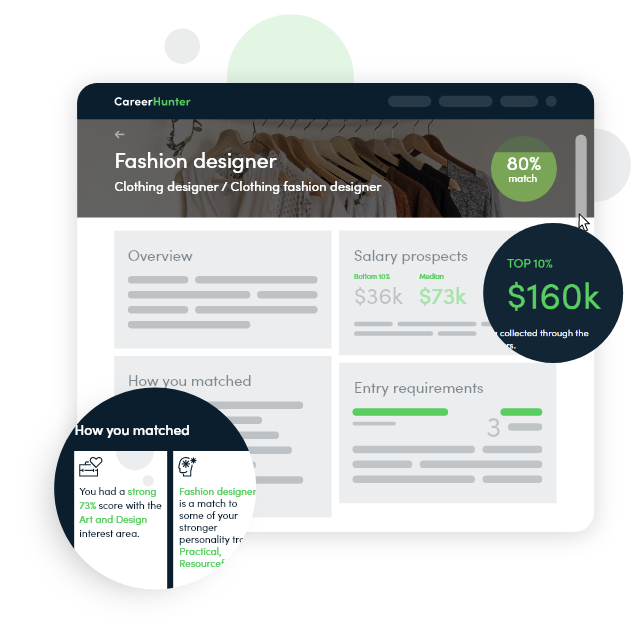The image depicts a web page from Career Hunter, displaying detailed career information for a Fashion Designer. At the top, a black header prominently features the Career Hunter logo in white and green text. Directly below the header, a back arrow is followed by the title "Fashion Designer," with a subtitle reading "Clothing Designer / Clothing Fashion Designer" in white text.

A green circular icon indicates an 80% match for the user's compatibility with this career. Further down, there are several sections: "Overview," "How You Matched," and "Salary Prospects." The salary prospects range from $36,000 to $73,000, noting that the bottom 10% earn $36,000, while the median salary is $73,000. An additional black circle with green text highlights that the top 10% can earn up to $160,000.

Another pop-up circle explains the user's matching criteria: "You had a strong 73% score with our InDesign interest area. Fashion Designer is a match to some of your stronger personality traits." Overall, the page provides a comprehensive overview, detailing salary expectations and personalized matching information for a career in fashion design.